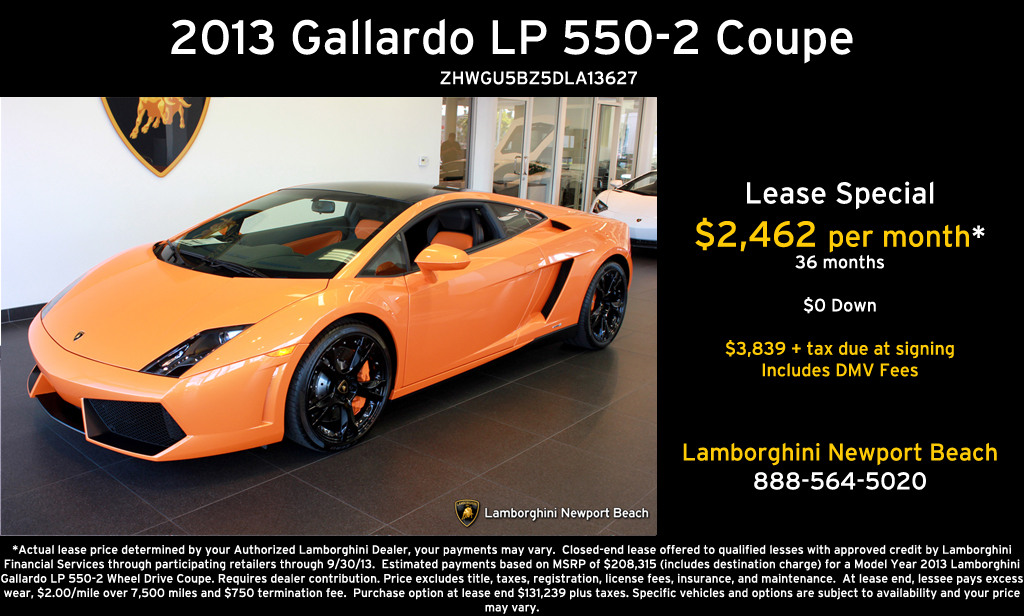The image showcases an advertisement for an orange 2013 Lamborghini Gallardo LP 550-2 Coupe, prominently placed indoors. Along the top of the image, a black border in white text details the car’s model and VIN: "2013 Gallardo LP 550-2 Coupe, ZHWGU5BZ5DLA13627." On the right side of the border, text promotes a lease special, highlighting in white "Lease Special" and in orange "$2,462 per month, 36 months." Further details include "36 months, $0 down" and "$3,839 plus tax due at signing, includes DMV fees," also emphasized in orange. The dealership, Lamborghini Newport Beach, is named below in orange text, followed by their contact number in white: "888-564-5020." The advertisement, with its detailed financial terms and fine print disclaimers at the bottom, underlines a high-end financing offer for this luxury sports car.